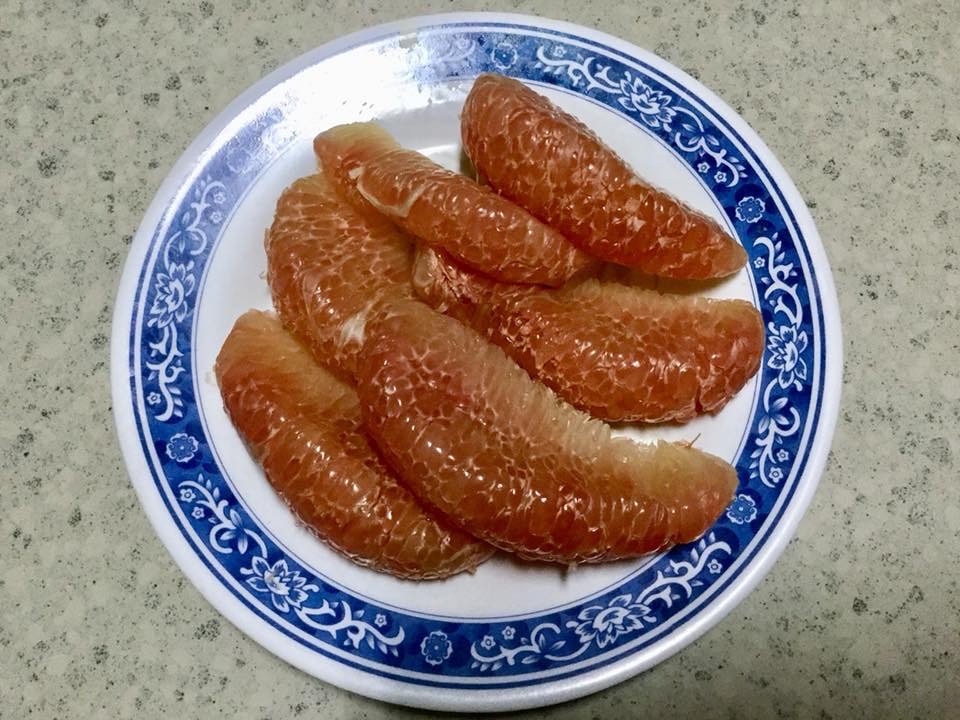The photo features a white circular plate adorned with a blue floral-patterned rim, sitting on a light gray granite or marble-like tabletop. The plate showcases six large, crescent-shaped slices of a mysterious food item, exhibiting a dark orange to brownish hue. The slices are arranged in an overlapping manner, creating a detailed and textured appearance that suggests a slick, possibly scaly surface, adding to the intrigue. A slight gleam of light, likely from a camera flash, highlights one corner of the plate, enhancing the visual contrast. Overall, the image is zoomed in, emphasizing the size and texture of the slices which could be baked apple slices, some type of fruit, or perhaps even a seafood delicacy.